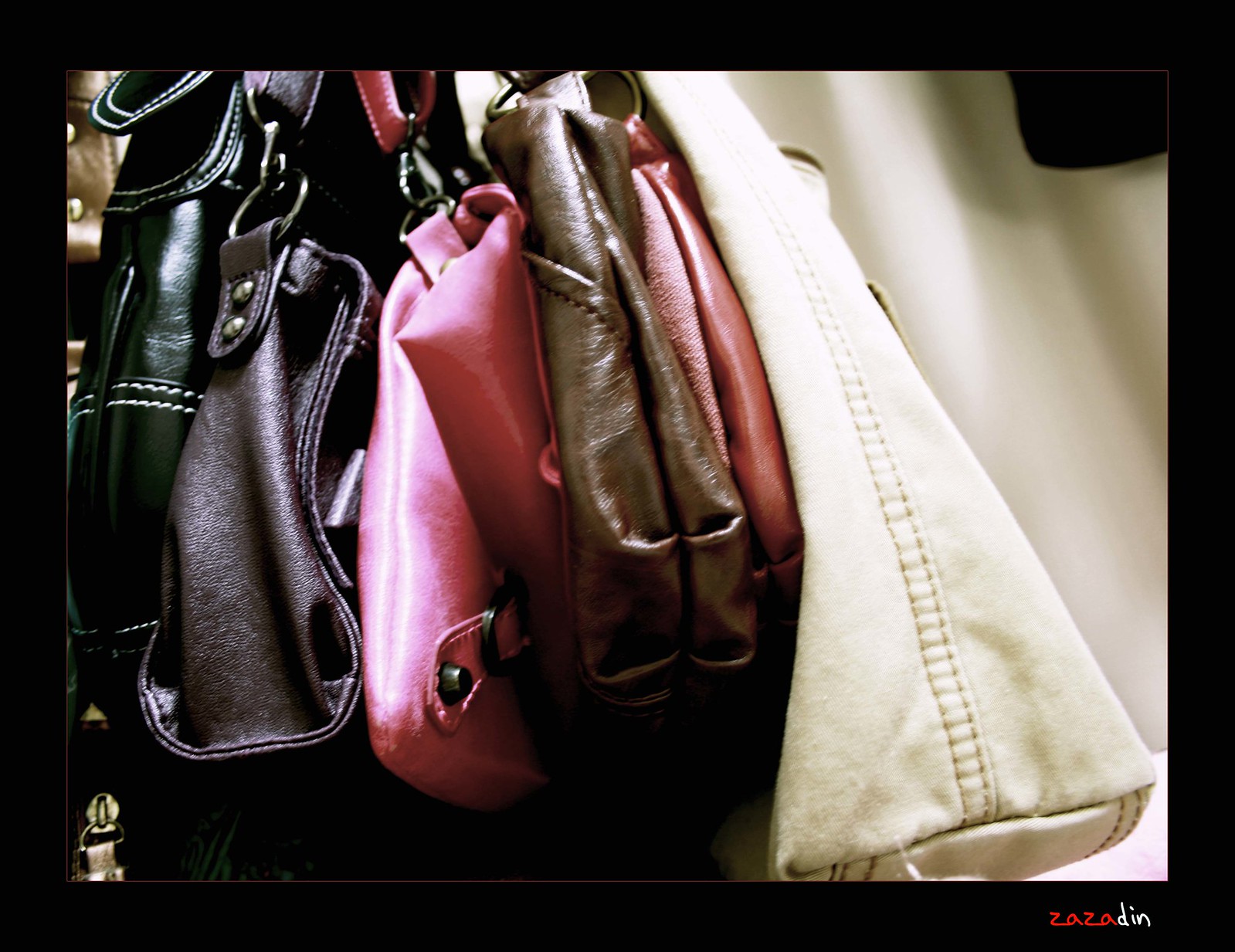The image is a detailed close-up photograph of seven distinct women’s handbags, appearing as if they're hanging from an unseen rack. From left to right, the first handbag is a shiny black leather with white stitching. Next is a deep brown or possibly dark purple bag, followed by two pink handbags, with the second pink one having black metal elements. The fifth bag is a medium brown leather, and the sixth is a reddish-brown leather bag. On the far right, there's an off-white or cream-colored canvas bag with beige stitching. The handbags are shown in a tightly packed arrangement, and the photograph is framed in black. At the bottom right corner of the image, “Zazadin” is written, with "Zaza" in red font and "Din" in white font. The background on the right side of the image is a white wall or a piece of fabric.